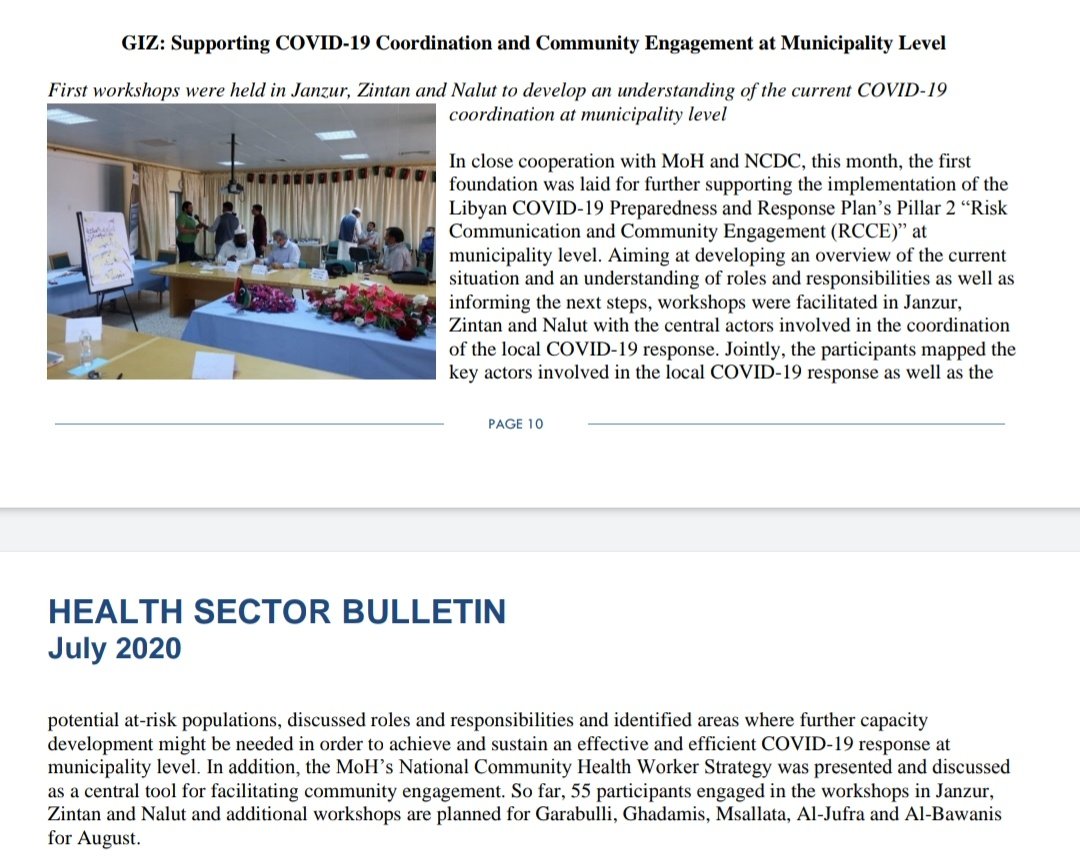The image captures a group of individuals seated around a table in a room, intently focusing on a whiteboard with writing on it. The text on the whiteboard signifies the GIZ’s support in COVID-19 coordination and community engagement at the municipality level. The first workshops, facilitated in Jamzor, Zintan, and Nalut, aimed to evaluate and comprehend the current state of COVID-19 coordination within municipalities.

In collaboration with the Ministry of Health (MOH) and the National Center for Disease Control (NCDC), these workshops represent the foundational steps toward enhancing the implementation of the Libyan COVID-19 Preparedness and Response Plan, specifically focusing on Pillar 2: risk communication and community engagement. The objective was to outline the current landscape and clarify roles and responsibilities, setting the stage for subsequent efforts.

The participants, composed of central figures in local COVID-19 response coordination, engaged in detailed mapping of key actors involved in the pandemic response. The caption references page 10 of the Health Sector Bulletin from July 2020.